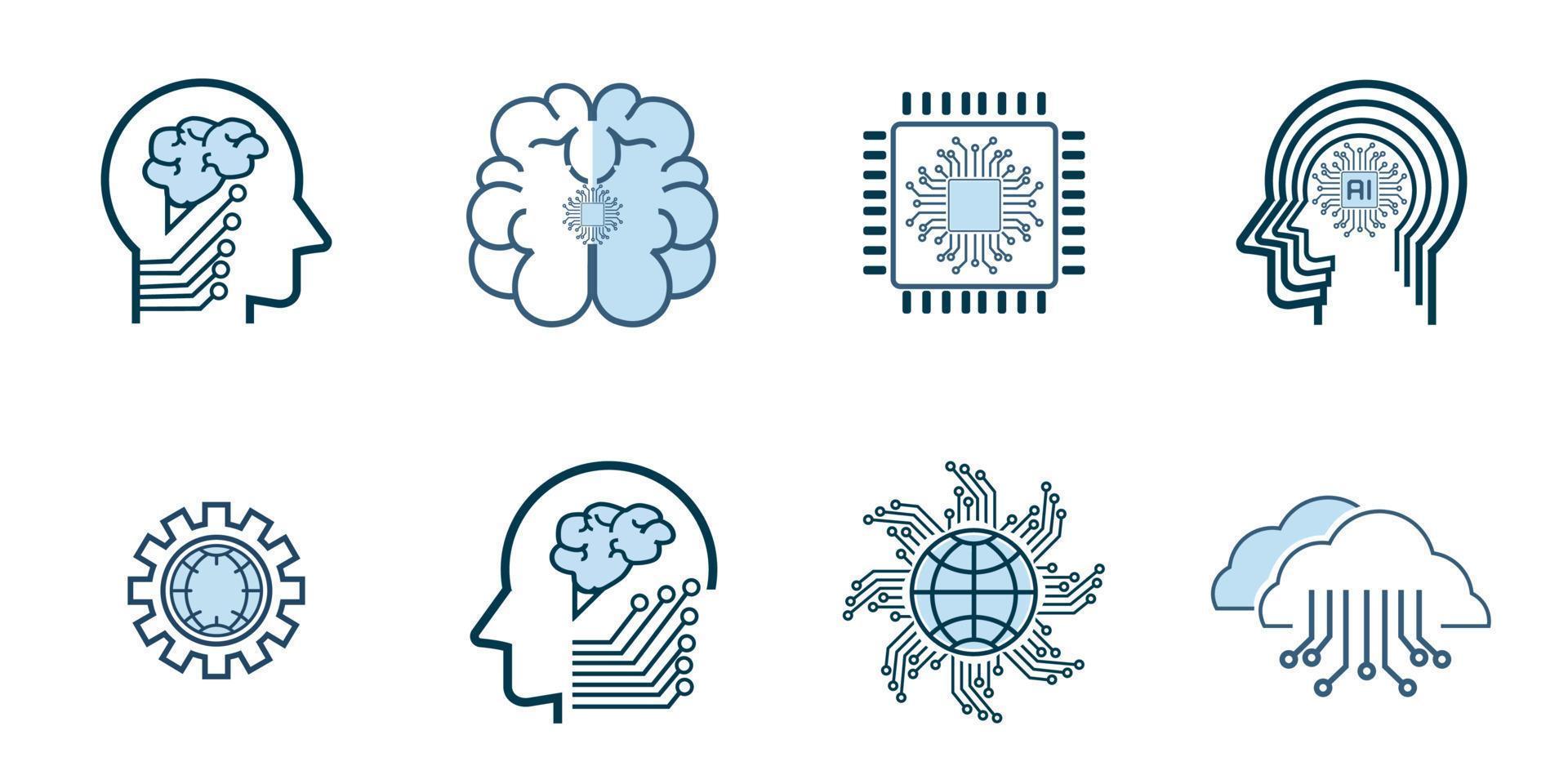The image is a color illustration oriented in landscape format, featuring eight diagrams arranged in two rows of four. Each diagram is a simple line art drawing primarily in light blue and black on a white background, with some incorporating silhouettes of human heads. These heads typically feature internal views of the brain highlighted in blue or white. 

Starting from the top left, the first diagram shows a head with lines emanating from the back of the neck towards the brain area, colored blue. The second diagram to its right reveals a more detailed view of the brain's two hemispheres, with one half colored blue and the other white. The third diagram is a schematic resembling a transistor, with lines extending from a central square in multiple directions. Moving right, the fourth diagram depicts another head silhouette with various lines spreading out to different head sections.

On the bottom row, directly beneath the first head, there is an illustration of a gear, resembling a flywheel. The subsequent diagram to the right indicates signals being transmitted from the brain to a circular structure surrounded by cells. Further right, a depiction includes two cloud shapes, one white and one blue, with the white cloud featuring lines and hollow dots extending outwards. The final diagram on the bottom right features repetitive circuitry elements paired with the aforementioned cloud shapes.

Overall, the illustration seems to portray the development and transmission of ideas or signals within the brain, extending through various schematic representations and abstract forms, all set against a minimalist white background.